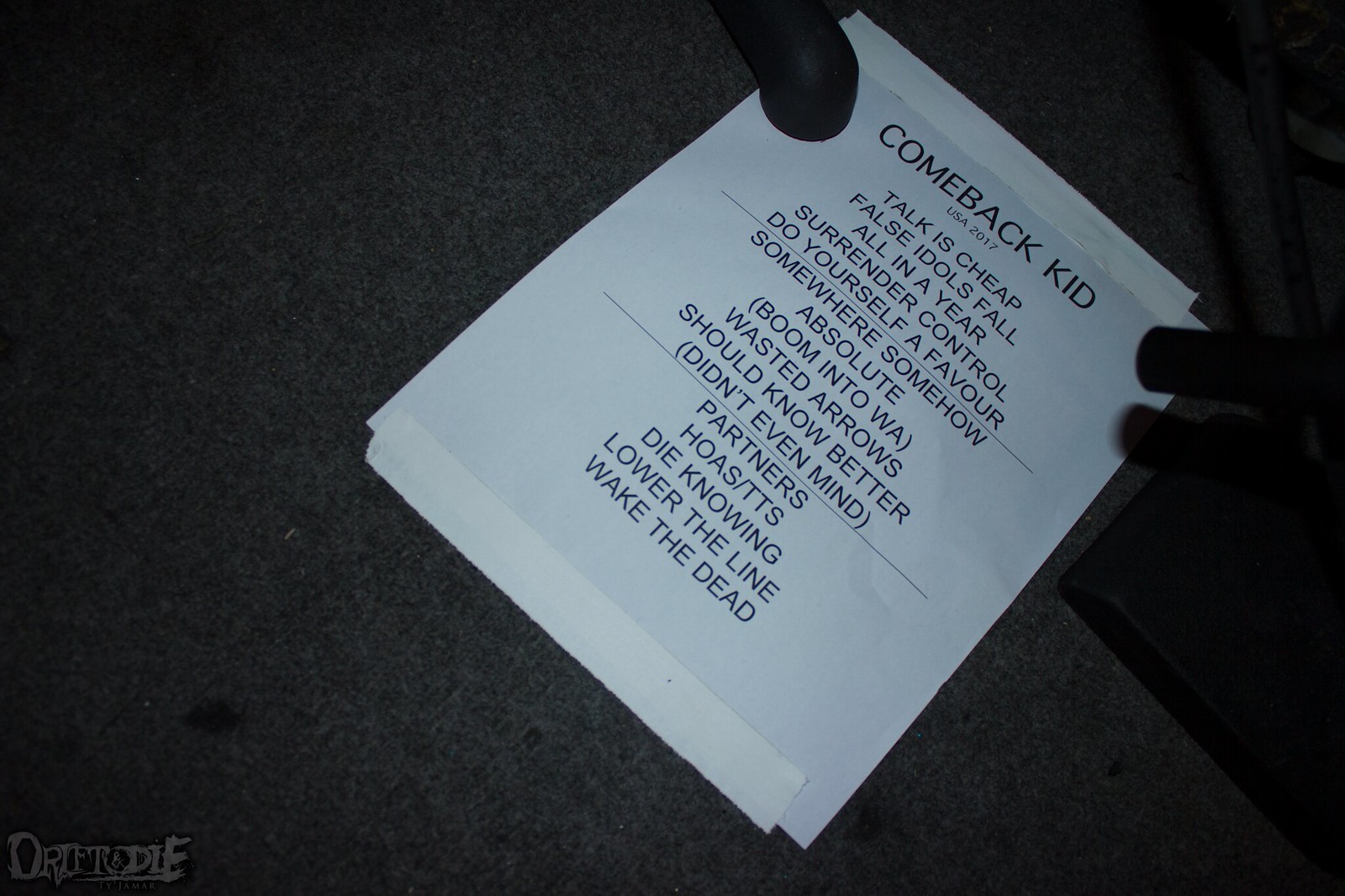The image is a photograph of a white piece of paper, affixed to a grey felt surface, likely a bulletin board or wall, using strips of white tape at the top and bottom. The paper appears slightly angled, with its top right corner pointing towards the top of the photograph and the bottom left corner pointing downwards. There is a noticeable hole in the upper left corner, suggesting the paper might have been in a binder or similar. The paper features multiple lines of black text, predominantly centered on the page. At the top, it reads "Comeback Kid USA 2017," followed by a series of what seem to be titles or statements: "Talk is Cheap," "False Idols Fall," "All in a Year," "Surrender Control," "Do Yourself a Favor," "Somewhere, Somehow," "Absolute," "Boom into the Wall," "Wasted Arrows," "Should Know Better," and "Don't Even Mind." Further down, additional statements include "Partners," "H.O.A.S.T.T.S.," "Die Knowing," and appear to cap off with "Wake the Dead." The text is printed in black ink, and there might be a watermark or some additional text reading "Drifter Die" on the bottom left of the paper.